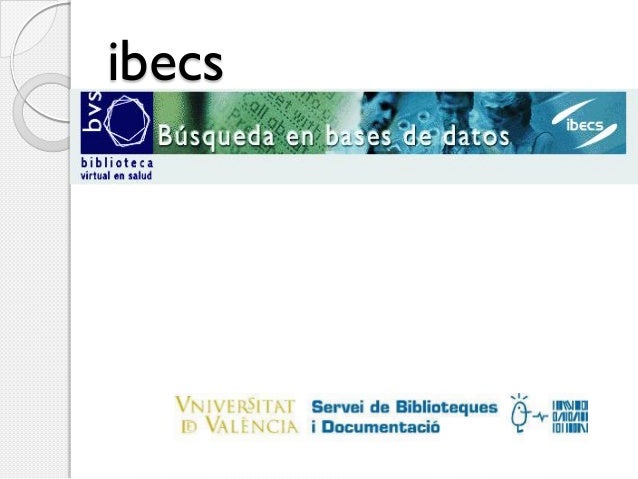This image appears to be a poster or a cover page and is predominantly in Spanish. It features a white background with a vertical gray border on the left side, which includes decorative elements resembling circles and semi-circles. In black text at the top left, it prominently displays the acronym "IBEC," written as I-B-E-C-S.

Below this, there's a header section incorporating colors such as blues and greens, and possibly an image depicting people in an office setting reviewing documents. Within this multicolored header, the acronym "BVS" and the words "BUSQUEDA EN BASES DE DATOS" are visible in white text. Additionally, "IBEC" appears again within a design that includes flared white lines resembling comets.

Subsequent to this, on a gray background with blue text, the phrase "BIBLIOTECA VIRTUAL EN SALUD" is written, referring to a virtual health library. Towards the bottom of the image, there's significant white space and then more text, indicating "UNIVERSITAT ID VALENCIA SERVEI DE BIBLIOTEQUES DOCUMENTACIÓ," along with a small graphic of a figure, possibly a bird, in front of a bookshelf. The overall design suggests it is related to library services and documentation from the University of Valencia.